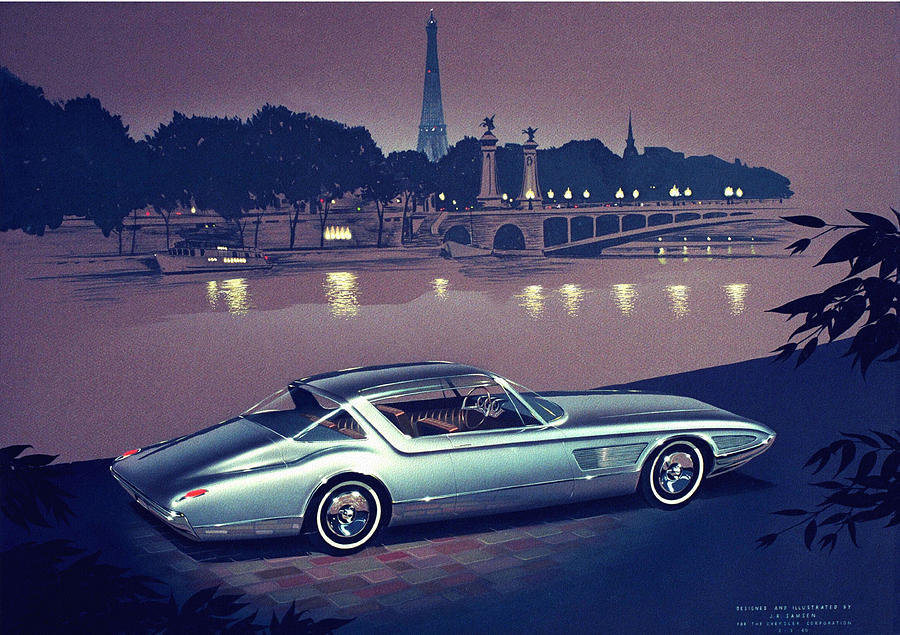This illustration, possibly a vintage-themed postcard or poster, depicts a classic and meticulously detailed car, potentially one of the first Corvettes, parked along a serene riverbank in Paris, France. The car, shining in a metallic bluish-gray hue, features rigid leather seats, an enormous steering wheel, and chrome bumpers that accentuate its antique charm. Notably, the taillights are striking red, positioned on either side of the trunk.

The backdrop of this scene is the iconic Eiffel Tower, partially shrouded in the mist, with a faint glow illuminating its structure. To the right, a bridge, possibly the famous Pont des Arts (Lock Bridge), stretches across the river, its lights reflecting beautifully in the water below. A sailboat, adorned with lights and carrying people, glides on the river, enhancing the picturesque setting.

Branches from nearby trees frame the scene, adding depth and a touch of nature to the cityscape. The rich reddish-brown tones of the landscape suggest it is either dusk or dawn, wrapped in a soft, dreamy fog. At the bottom right corner of the image, the artwork is signed by J.R. Timmons, contributing to its authenticity and artistic value.